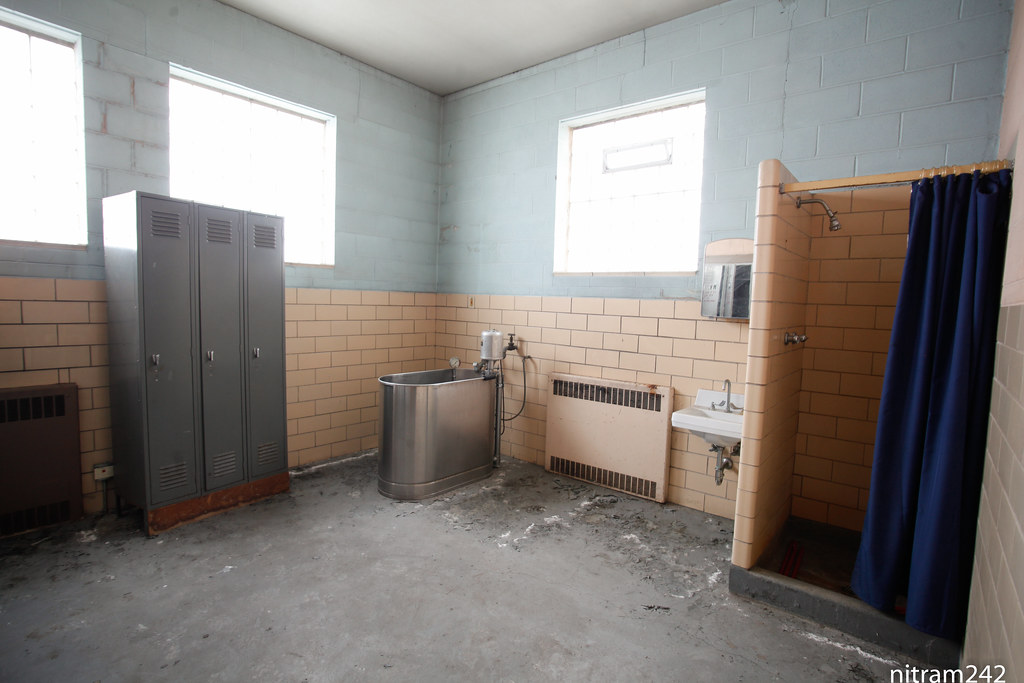This image captures a bathroom or locker room in an institutional setting such as a gym or school. The room features a gray concrete floor and cinder block walls, which are painted in two shades: a light grayish-blue on the top half and a beige or pinkish-tan on the bottom half. On the right side of the image, there is a stand-in shower with beige tiles and a dark blue curtain. Adjacent to the shower, on its left, is a small white ceramic sink.

Dominating the left side of the image are three gray lockers with air vents at the top and silver handles in the middle. Positioned between the shower and the lockers is a large radiating or heating unit, and another similar unit is visible on the left side of the room. In the corner stands an oval-shaped metal tub with some sort of device extending into it. The room is well-lit overall, highlighted by three large, bright windows at the top of the image, allowing daylight to spill in and illuminate the space.